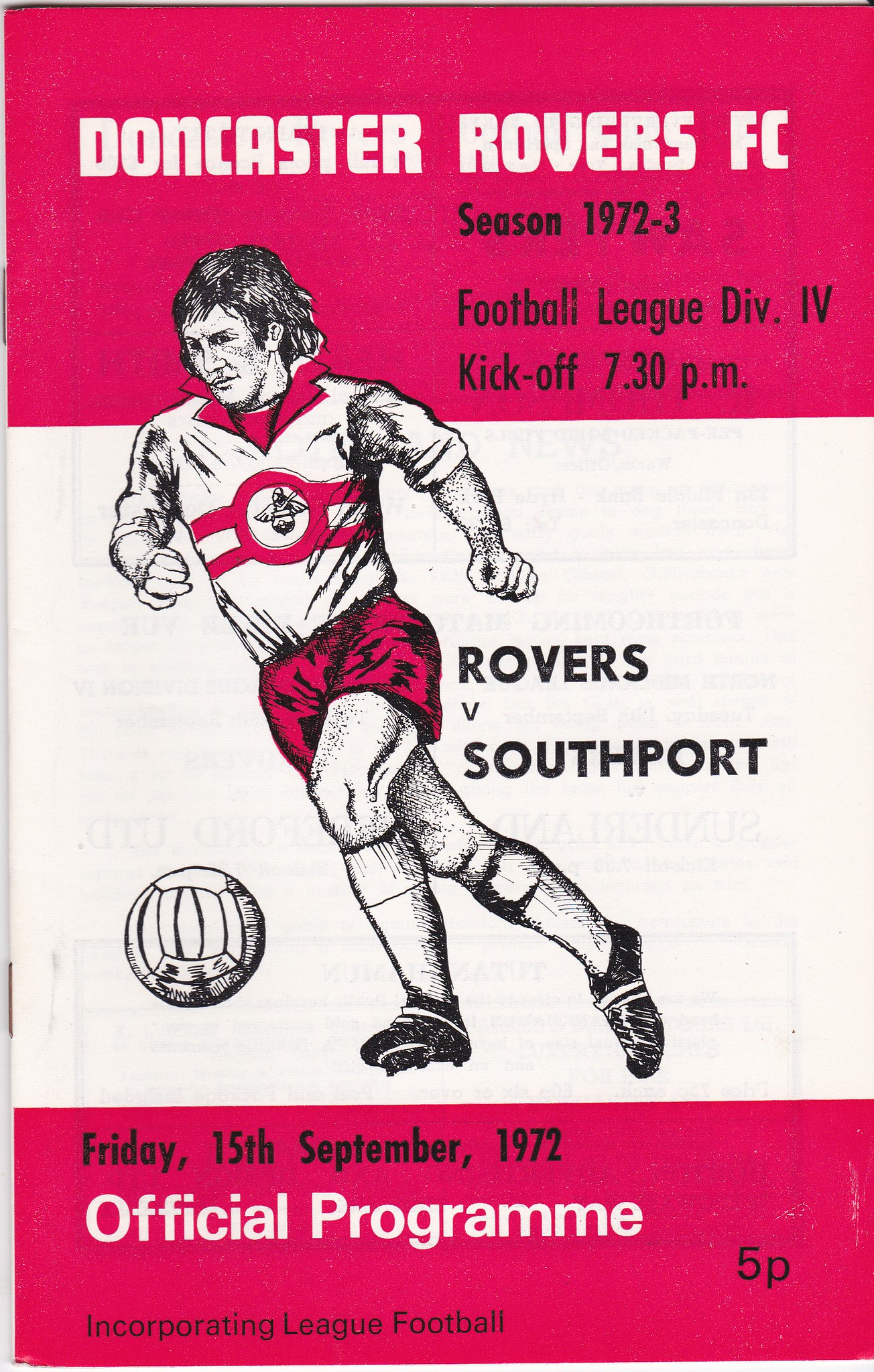The image depicts the front cover of an official program for a Football League Division 4 match, prominently featuring Doncaster Rovers FC. The title, "Doncaster Rovers FC," is set against a red background at the top, with the subtitle "Season 1972-3, Football League Division IV, Kickoff 7.30pm" in black text immediately below. The middle section has a white background showcasing an illustration of a soccer player in motion, poised to kick a ball at his feet. The player, donned in red shorts and a white shirt with red stripes and a red collar, is looking to his left, with his head and shoulders extending into the red section above. Adjacently, in black text, it states "Rovers v. Southport." The bottom quarter reverts to a red background and details "Friday 15th September 1972" in black, followed by "Official Program" in white text, and underneath, "Incorporating League Football 5P" in black. The cover effectively combines the excitement of the game with the essential information, making it a comprehensive memento for attendees.